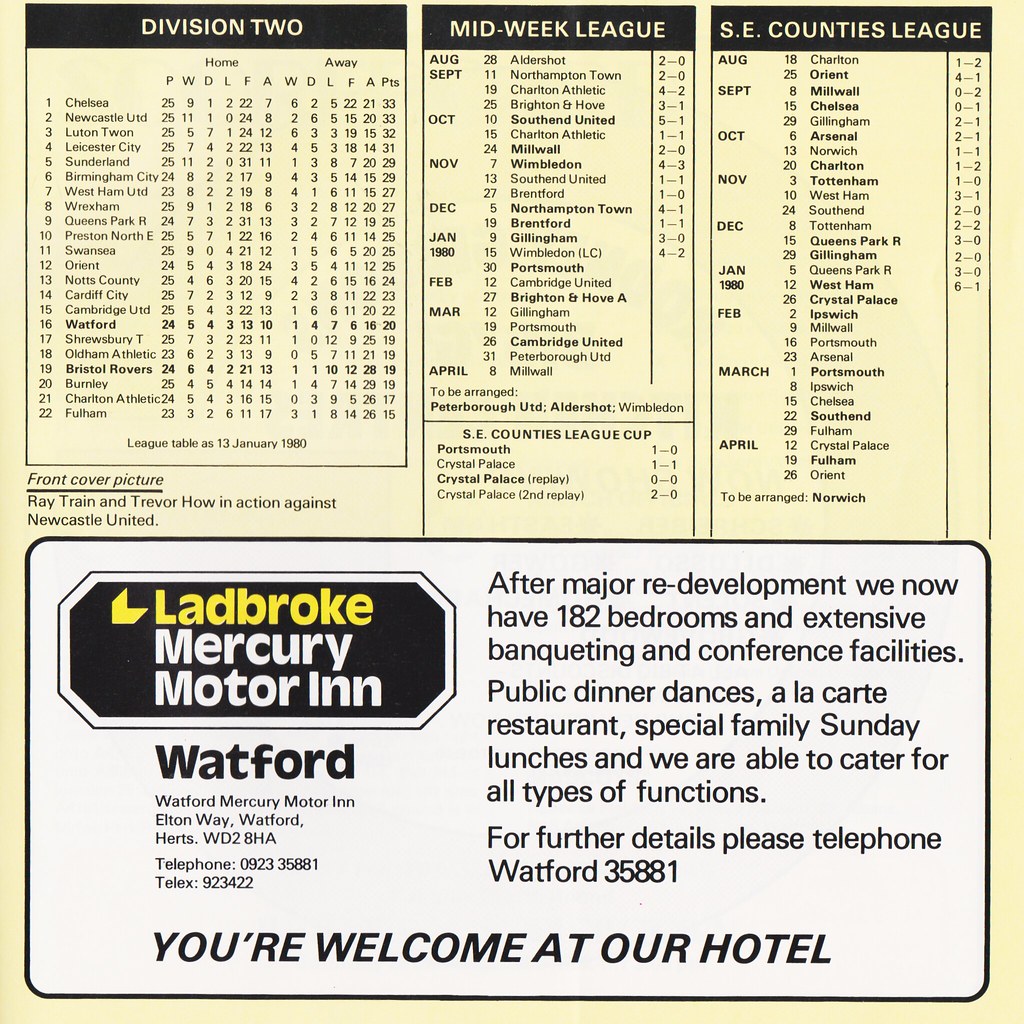The image features a perfectly square layout with a muted yellow background. The top half is divided into three vertical segments, each bordered by black headers against the yellow backdrop. The segments are labeled: Division II, Midweek League, and SE Counties League. 

- The Division II section displays a list of teams numbered 1 through 22, accompanied by charts detailing Home and Away game statistics.
- The Midweek League segment includes a schedule with dates, locations, and scores of various matches.
- Similarly, the SE Counties League segment also offers a schedule listing dates, locations, and scores.

Additionally, a small caption mentions a "front cover picture of Ray Train and Trevor How in action against Newcastle United."

The bottom half of the page features an advertisement for the Ladbroke Mercury Motor Inn. The white business card-style ad with black text highlights "Ladbroke" in yellow. It includes the address and a message: "You're welcome at our hotel." The ad also details the hotel's amenities, including 182 bedrooms, banqueting and conference facilities, public dinner dances, an a la carte restaurant, and special family Sunday lunches. For more information, it provides a contact number: Wadford 35881.